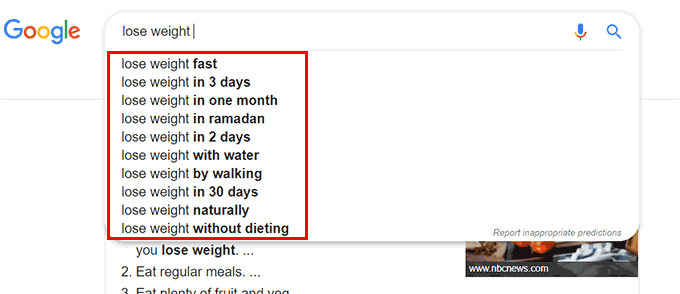Here's a detailed, cleaned-up, and descriptive caption for the image:

"A screenshot of a Google search results page with a distinct white background. In the top left corner, the iconic Google logo is prominently displayed, featuring an uppercase blue 'G', followed by two lowercase 'o's in red and yellow, a lowercase blue 'g', a lowercase green 'l', and a lowercase red 'e'. To the right of the logo is the search bar, containing the query 'lose weight'. Below the search bar, Google's autocomplete suggestions are visible, highlighted inside a red box. To the right of the search bar are the microphone and search icons. Further down the page, partial search results are listed, with the numbered section 1, 2, and a partially visible 3 due to the dropdown box. In the bottom right corner, a snippet from an NBC News article is featured."